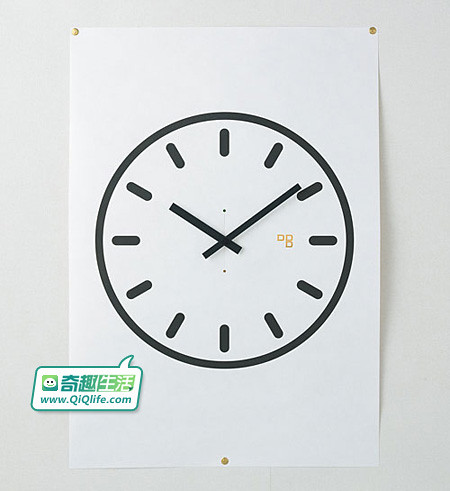In this minimalist image, a stark white wall serves as the backdrop for a single white sheet of paper fastened securely by thumbtacks. There are four thumbtacks in total: two at the top corners and one at the bottom center, with the fourth not explicitly mentioned but implied to be near the bottom. 

Centered on the paper is a simple clock illustration, created with black marker. The clock features a single bold circle and twelve small black lines indicating the hours. Two black hands, one for the hour and one for the minute, mark the time. To the left of the numeral three on the clock, three small gold squares add a touch of color and intrigue.

In the bottom left corner of the paper, there's a small text box containing Chinese characters, a smiley face, and a web address: www.QIQLife.com. This detail provides a cultural and digital connection to the otherwise simplistic and timeless design.